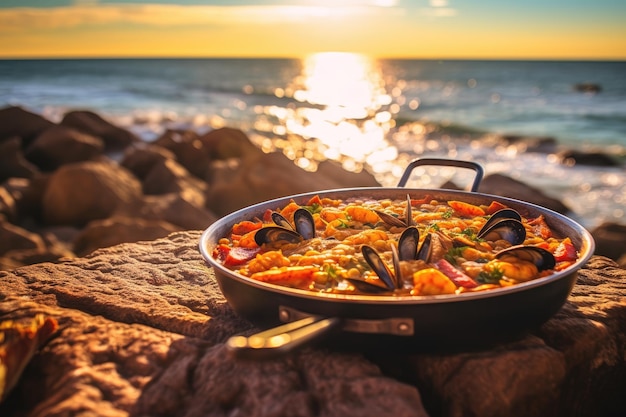In this image, we have a beautifully staged seafood dish presented in a rugged, natural setting by the beach at sunset. The dish, which seems to be a variant of gumbo or a seafood risotto, is rich in ingredients like mussels with black, open shells, shrimp, and sausage. There are hints of red from tomatoes and a mix of green vegetables, adding vibrant colors to the reddish-yellow sauce. The mixture sits in a black saucepan with a brushed metal rim and handles on either side, resting atop a rock. The background reveals a stunning, slightly out-of-focus ocean scene with the sun nearing the horizon, casting a glowing orange and yellow hue across the sky and water. This picturesque setting, complete with soft, blurred reflections off the ocean and additional rocks scattered along the shoreline, suggests the image might be designed for distinctive visual platforms like Instagram or a food blog.